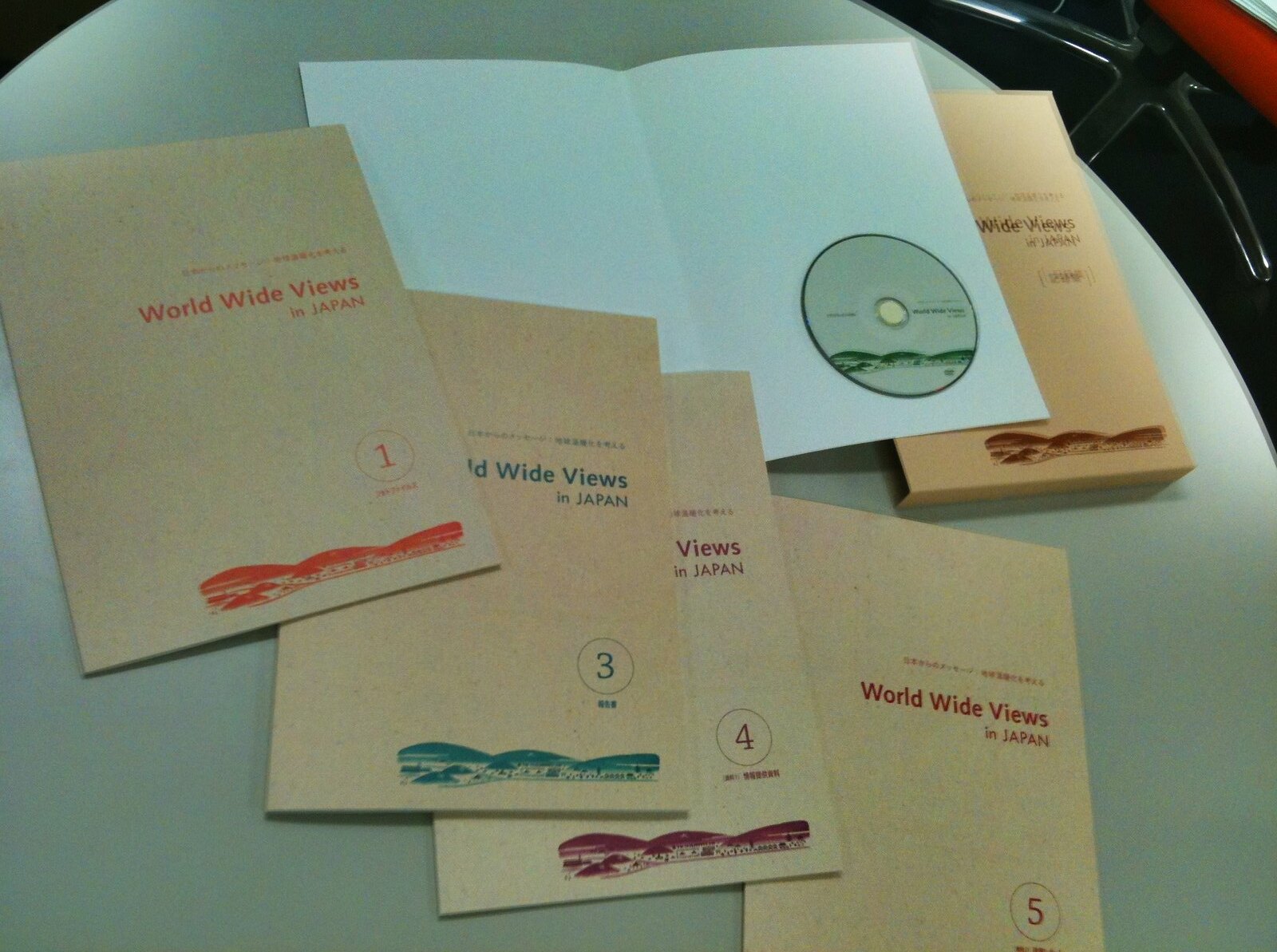In this image, we see a circular, white table cluttered with several pamphlets and booklets, which are part of a series titled "World Wide Views in Japan." These pamphlets are layered on top of one another in a way that their titles and numbering are visible—showcasing issues numbered 1, 3, 4, and 5. Each booklet features the same logo with mountain scenery at the bottom, in various colors like orange. Spread across the table and particularly noticeable in the center is an open booklet containing a CD or DVD on its right side, which has a picture of mountain scenery on it. The table is set indoors, likely in an office setting, as indicated by the partial view of a standard office chair with red seating and multiple legs with wheels in the upper right corner. Behind the table, there is a distinguishable black and red item, adding to the office-like ambiance. Tucked in the top right corner of the image, there seems to be a box intended for storing these folders. The setting appears clean and organized despite the multiple overlapping materials on display.